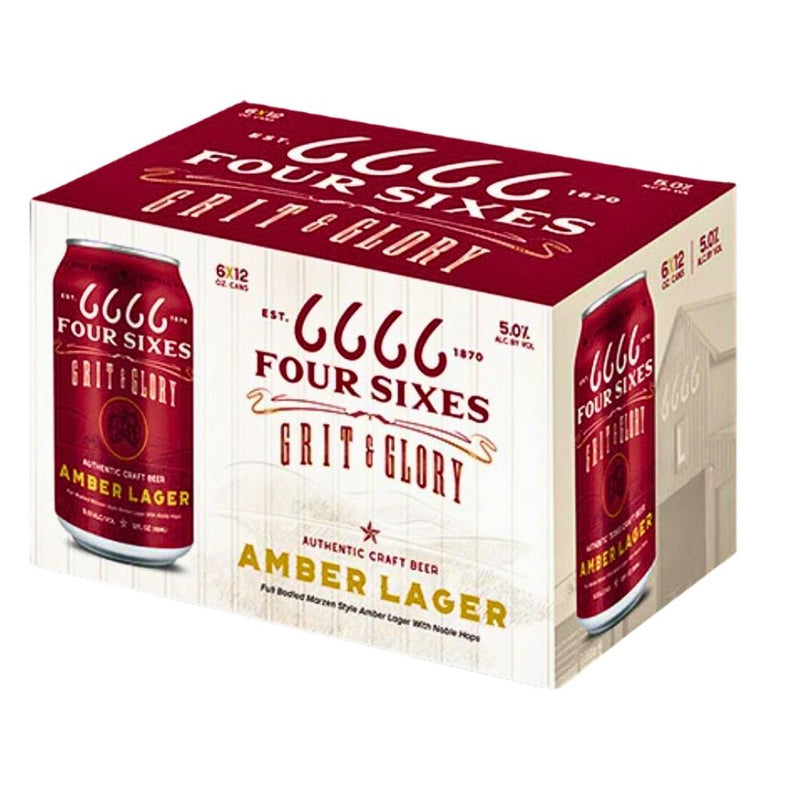The image displays a full-color photograph of a rectangular cardboard box containing Four Sixes Grit and Glory Authentic Craft Beer Amber Lager. The box, designed with a dark red top and white sides, prominently features the brewery's symbol "6666" on the top. The sides of the box showcase images of the red metallic beer cans, each labeled with "Four Sixes Grit and Glory Amber Lager" in gold lettering. One side of the box includes an illustration of a barn emblazoned with the four sixes symbol. The box holds twelve 12-ounce cans of beer.